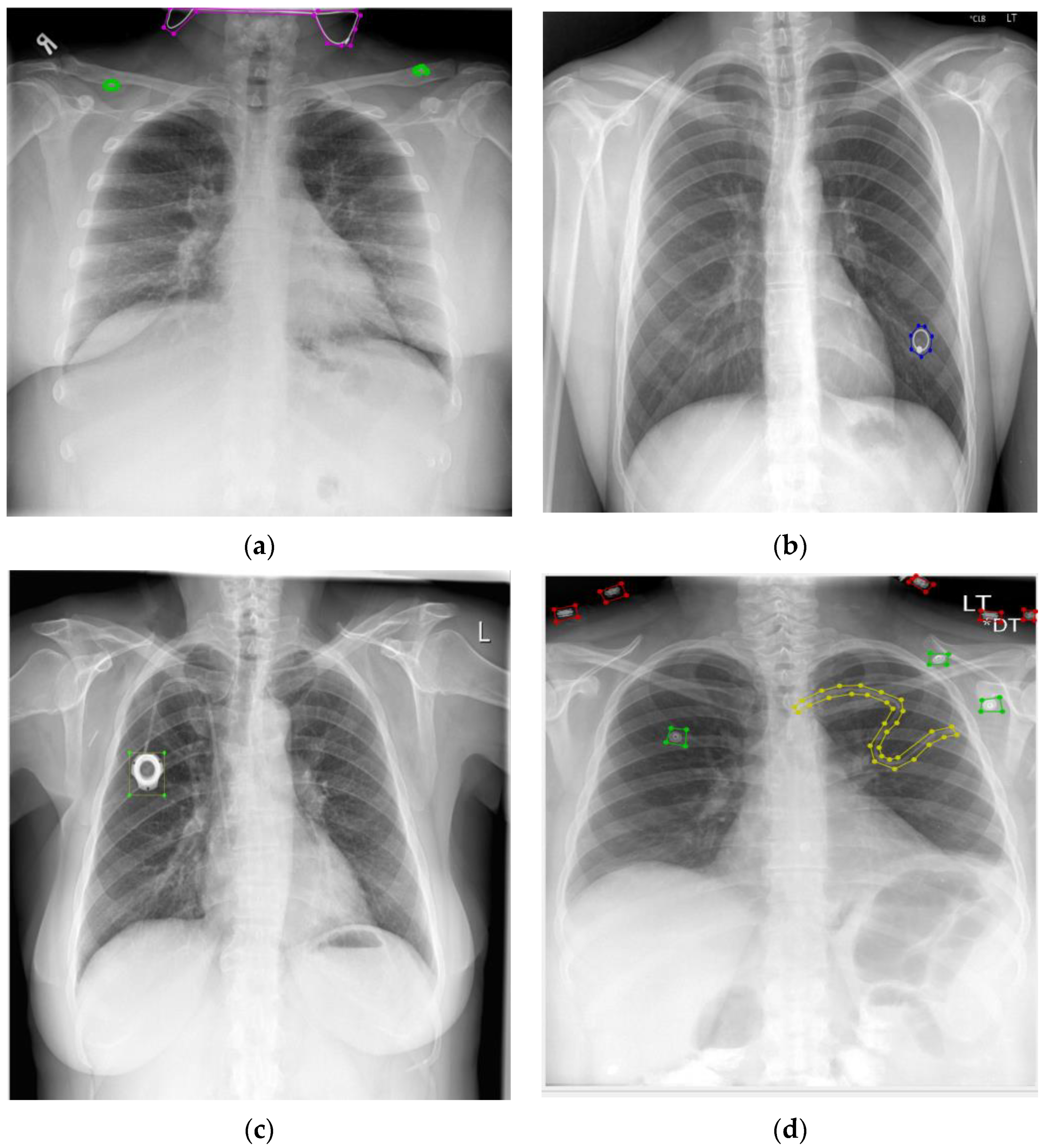This collection of four x-ray images, arranged in a 2x2 grid and labeled A, B, C, and D from top left to bottom right, provides a detailed view of the chest and lungs. Each black-and-white x-ray features colored markings to highlight areas of interest. 

1. **X-ray A**: Shows two small green dots marking each shoulder.
2. **X-ray B**: Contains a small blue dot located in the middle of the lower ribs.
3. **X-ray C**: Displays a white dot on the upper left rib, with what looks like a bolt-like shape going through the image.
4. **X-ray D**: Highlights a small green square on the upper left rib and a distinctive yellow, snake-like design in the upper right rib. This image also features two green dots near the upper right shoulder.

The consistent use of color-coded markers across these x-rays underscores critical areas and potential anomalies in the chest and ribs.